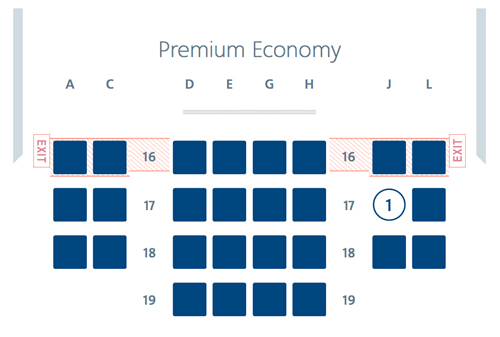The image is a detailed schematic layout of an aircraft's premium economy seating section on a white background. The seats are represented by blue squares arranged in rows and columns, identified by letters and numbers. At the top of the layout, gray text labels the section as "Premium Economy." 

The seat rows are labeled A, C, D, E, G, H, J, and L, with noticeable gaps where the letters B, F, and K are absent. On the far left, rows A and C each contain three seats per row. Following these, there is a numbered aisle space with the numbers 16, 17, 18, and 19. 

Continuing from left to right, the layout comprises four columns of seats identified as D, E, G, and H, forming four complete rows of seats. Adjacent to these, separated by another aisle, are the final two columns labeled J and L.

Notably, red exit signs are visible across the 16th row, indicating the emergency exits. This row marks the beginning of all columns, from A through L, enhancing the safety information within the seating schematic.